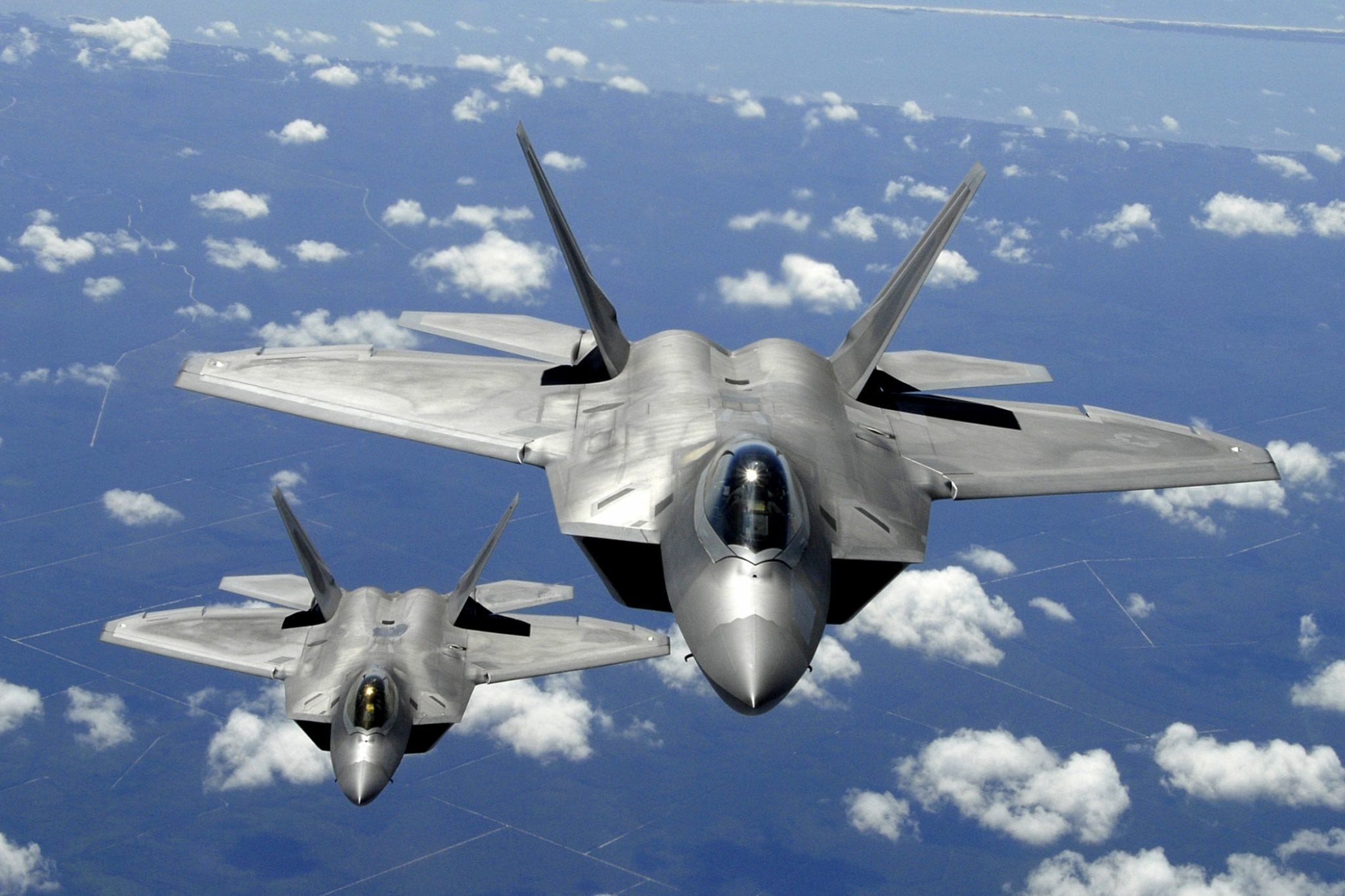This color photograph captures two silver-gray F-22 Raptor fighter jets flying through a light blue sky dotted with wispy, thin white clouds. The perspective is from another aircraft, looking back toward the approaching jets. The central jet is prominently featured with broad wings and two vertical stabilizers, and a black cockpit that does not reveal the pilot inside. Below and to the left of the primary jet, another similar fighter plane can be seen in flight. The sky and faint outlines of the landscape below provide a slightly dull backdrop, emphasizing the sleek, powerful design and formation of the military aircraft in this striking air-to-air image.